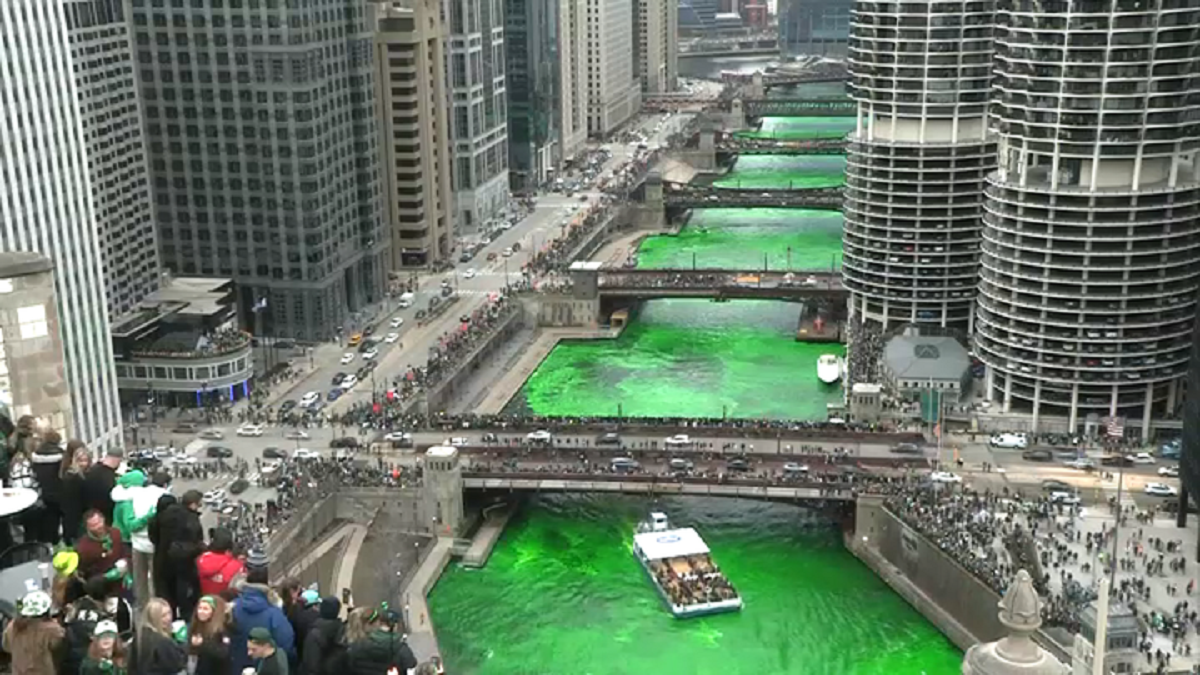This photo captures a vibrant scene of the Chicago River dyed bright green, a tradition for St. Patrick's Day celebrations. Tall skyscrapers and cylindrical towers with balconies line both sides of the river, combining to form the iconic cityscape. The upper sections of the buildings are adorned with glass windows, while the lower sections feature parking lots. Numerous bridges span the green-dyed water, crowded with people dressed in winter garb, hinting at the chilly weather. On the river, a large, partially-roofed sightseeing boat navigates the water, full of people admiring the grand architecture of the city. The bustling sidewalks and streets further showcase the lively atmosphere unique to Chicago during this festive occasion.